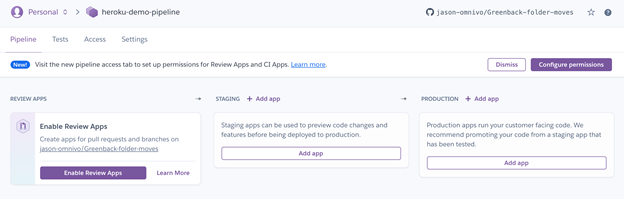This image is a blurry horizontal screenshot displaying a Heroku pipeline interface. At the top, there's a horizontal light gray bar featuring a label "Personal" in purple on the left-hand side, and references to "Heroku Demo Pipeline." On the right-hand side, it mentions "json.omnivo greenback-folder-moves."

Beneath the gray bar, a white strip extends horizontally, presenting options labeled "Pipeline," "Tests," "Access," "Settings," and "New." Below this, there's a notification suggesting users visit the "New Pipeline Access" tab to set up permissions for review apps and CI apps, with an option to "Learn More." To the right of this notification, there are two buttons: a dismiss button and a purple "Configure Permissions" button.

Further down, a horizontal gray box contains three white boxes arranged horizontally. 
- The first white box is for enabling review apps and provides an option to create apps for pull requests and branches on "json.omnivo greenback-folder-moves." It includes options to "Enable Review Apps" and "Learn More."
- The second white box explains that staging apps can be used to preview code changes and features before deploying to production.
- The third white box details that production apps run customer-facing code and suggests promoting code from a thoroughly tested staging app. Both the staging and production boxes feature "Add App" buttons.